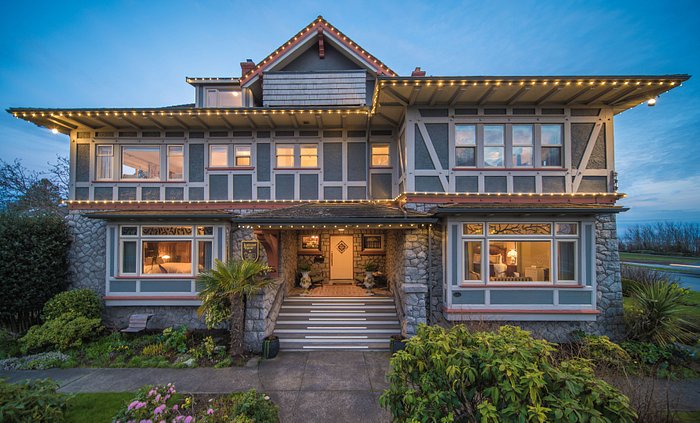This image depicts an elegant, potentially CGI-rendered two-story house at twilight. The structure exudes a sense of surreal perfection, combining elements of stonework on the lower level and possibly wood or hardy plank on the upper level. The house's façade features large, illuminated windows that allow a warm glow to emanate from within. The front porch is supported by stone columns, leading to a front door accessed via a series of six or seven concrete steps. The exterior is adorned with festive bulb and string lighting that outlines the roof and edges of the house, emitting a yellowish glow. The neatly landscaped yard includes a small palm tree, green bushes, and pink flowers, enhancing the inviting atmosphere. In the backdrop, a serene coastal setting unfolds with clear views of blue water, leafless trees, and a partially clouded sky, reinforcing the tranquil scene captured either at dawn or dusk.